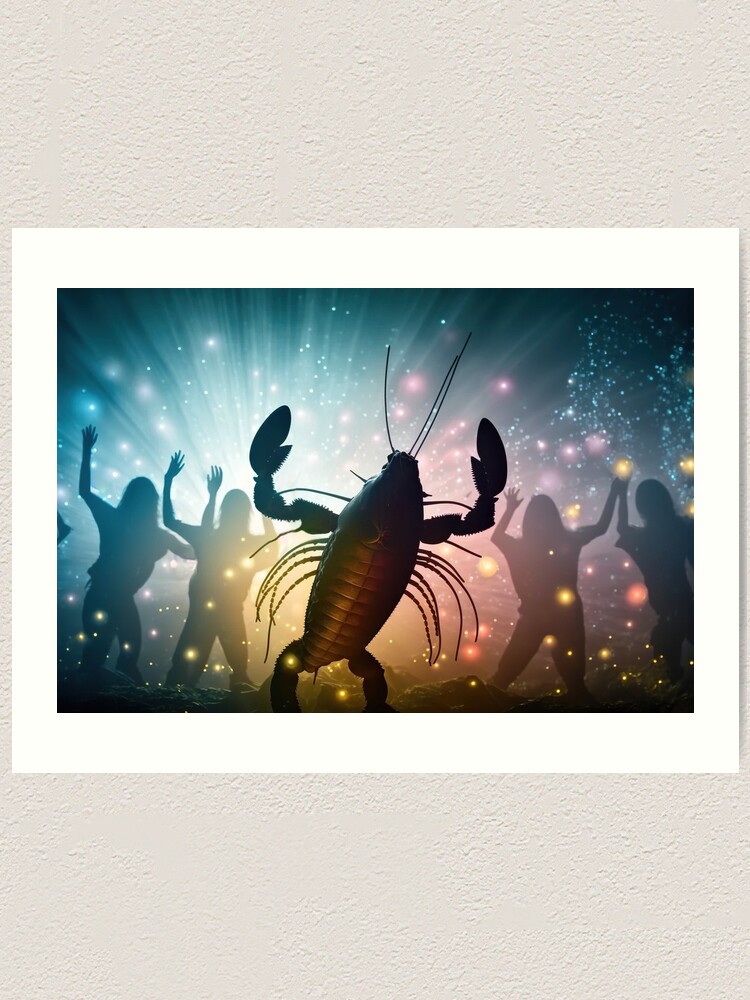This detailed image depicts a vibrant dancing lobster with its claws raised in the air, set against a backdrop of dazzling lights and fireworks. Surrounding the lobster are silhouettes of what appear to be four dancers, possibly cavemen or Bigfoot, with their arms raised and fingers apart as they join in the dance. The background is illuminated with a sparkling array of colors, including blue, yellow, pink, red, and purple, which create the effect of fireworks amid a glimmering, starry sky. A prominent blue shining light stands out among the colorful sparkles, and tiny glitter accents the right side. The edges of the image are very dark, especially in the four corners, adding a dramatic contrast to the bright central scene. The piece is rectangular with a white border and hangs on a cream-colored, textured wall. The entire composition exudes a lively, celebratory atmosphere, capturing a joyous moment in time.